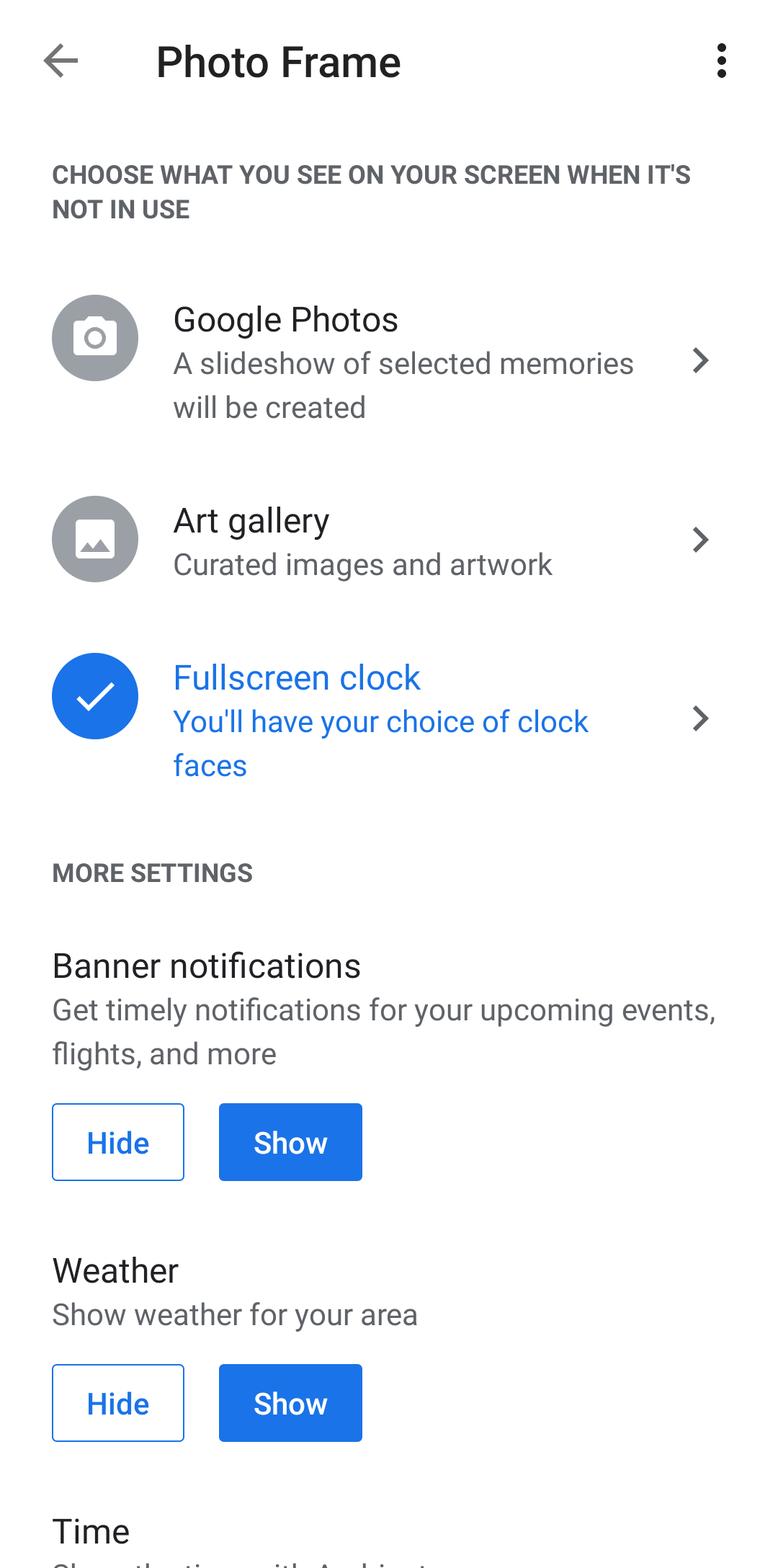This screenshot captures a settings page within a photo application. At the top, there is a "Photo Frame" label and a back button in the upper left corner. Directly beneath the title, caption text reads, "Choose what you see on your screen when it's not in use."

The settings options are displayed in three distinct rows:

1. **Google Photos**: Described further with the text, "A slideshow of selected memories will be created."
2. **Art Gallery**: Accompanied by the text, "Curated images and artwork."
3. **Full-Screen Clock**: This option, marked with a checkmark and highlighted in blue, states, "You'll have your choice of clock faces."

Below these primary options, another section labeled as "More Settings" appears, featuring additional configurable items:

- **Banner Notifications**: This toggle option, currently set to "Show," allows the user to receive timely notifications for upcoming events, flights, and more.
- **Weather**: Also set to "Show," this option displays the weather for the user's area.
- **Time**: This section provides a hide/show toggle, but the current selection is unclear as the screen is cut off.

This detailed summary provides a comprehensive understanding of the available settings and options within this particular photo application screen.